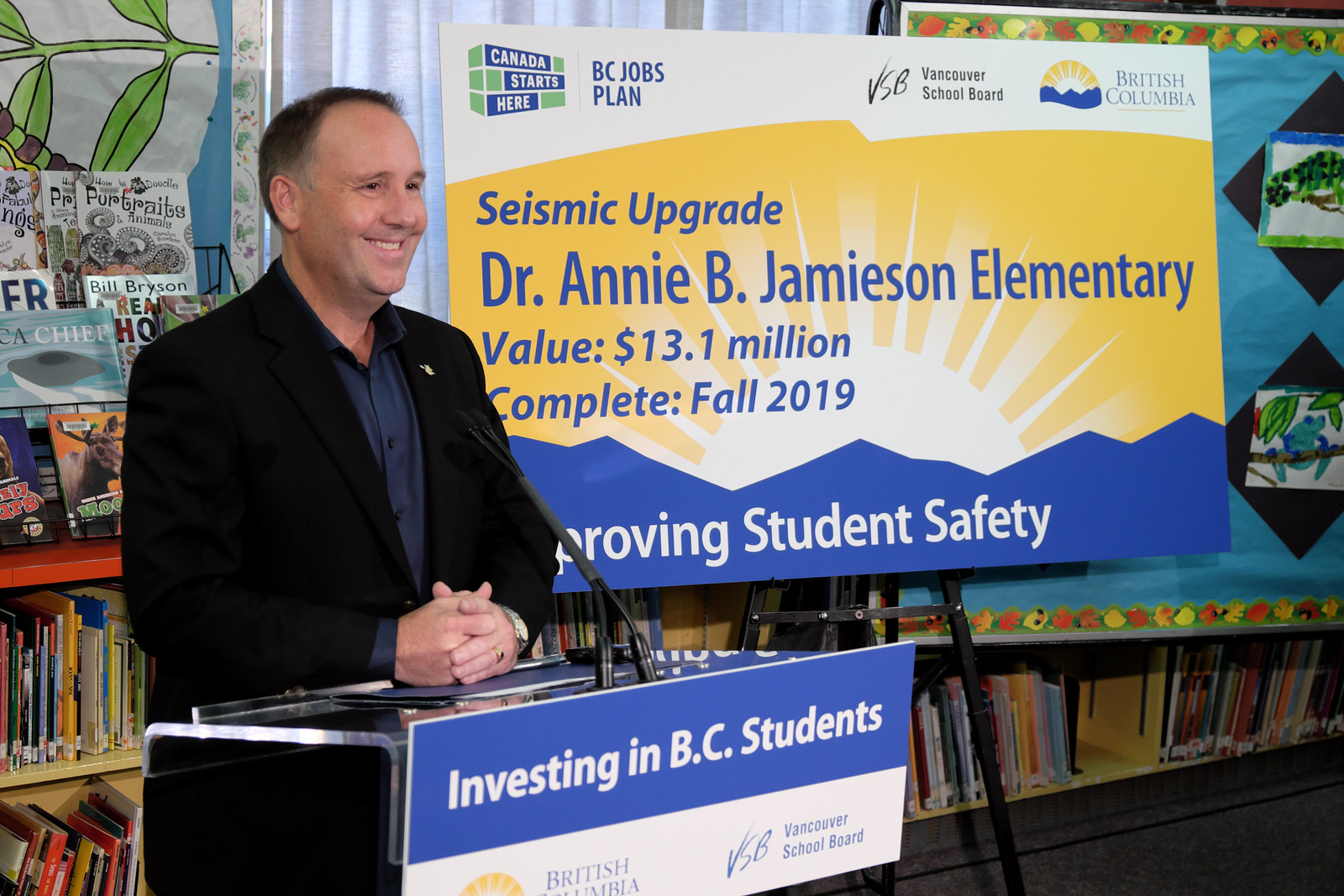In a brightly lit school library, a man in a black suit stands at a podium, hands folded politely in front of him and smiling as he poses for a photograph. He is preparing to give a talk about school improvements. The podium bears a sign with the text "Investing in BC Students" and "Vancouver School Board" in white. Behind him, shelves filled with children's books and colorful drawings, likely created by students, decorate the wall. To his right, a large sign details a significant project: "Seismic Upgrade, Dr. Annie B. Jamieson Elementary, Value $13.1 million, Complete Fall 2019, Improving Student Safety," part of the BC Jobs Plan. This suggests a substantial investment aimed at enhancing the school's infrastructure for better student security.